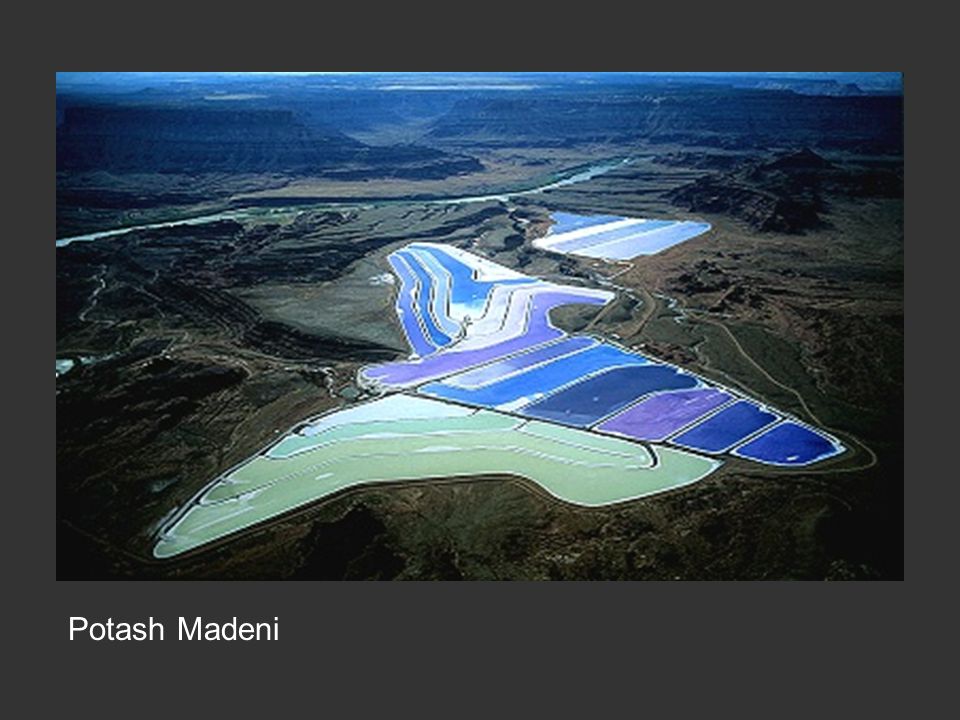This is an aerial photograph bordered by a thick gray frame, with the bottom portion particularly thick and a dark gray background. In the lower left corner of the frame, the words "Potash Madini" are displayed in white. The photograph itself captures a somewhat mountainous landscape with green areas and distinct mountains in the background. The foreground reveals a peculiar and artificial scene: sections of the land are covered with tarps or colored panels. The nearest section features a vivid green tarp, while other segments display varying shades of blue and purple, arranged in a pattern that stretches into the distance. These panels are divided into different sections, creating a visually striking contrast against the natural surroundings, reminiscent of the shape of an airplane with the 'nose' and 'body' in green and the 'tail' in blue tones.